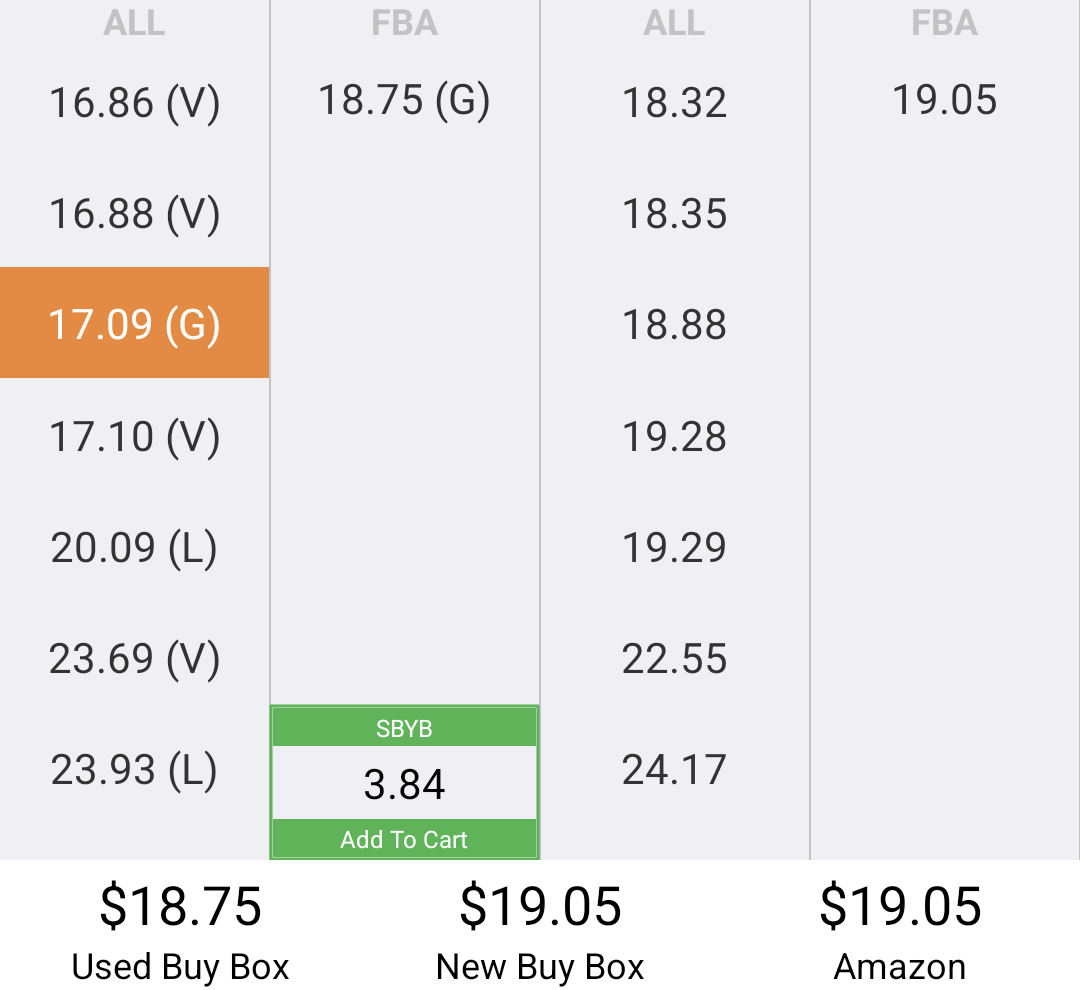This graph presents a comparative analysis of the prices for a certain product, possibly trading cards or a similar collectible item. The graph showcases three pricing options: a used box priced at $18.75, a new box available for $19.05, and the same new box listed on Amazon for $19.05. The detailed numerical data visually represent the minimal price difference between purchasing a new box directly or through Amazon, while highlighting a slight cost savings when opting for a used box.